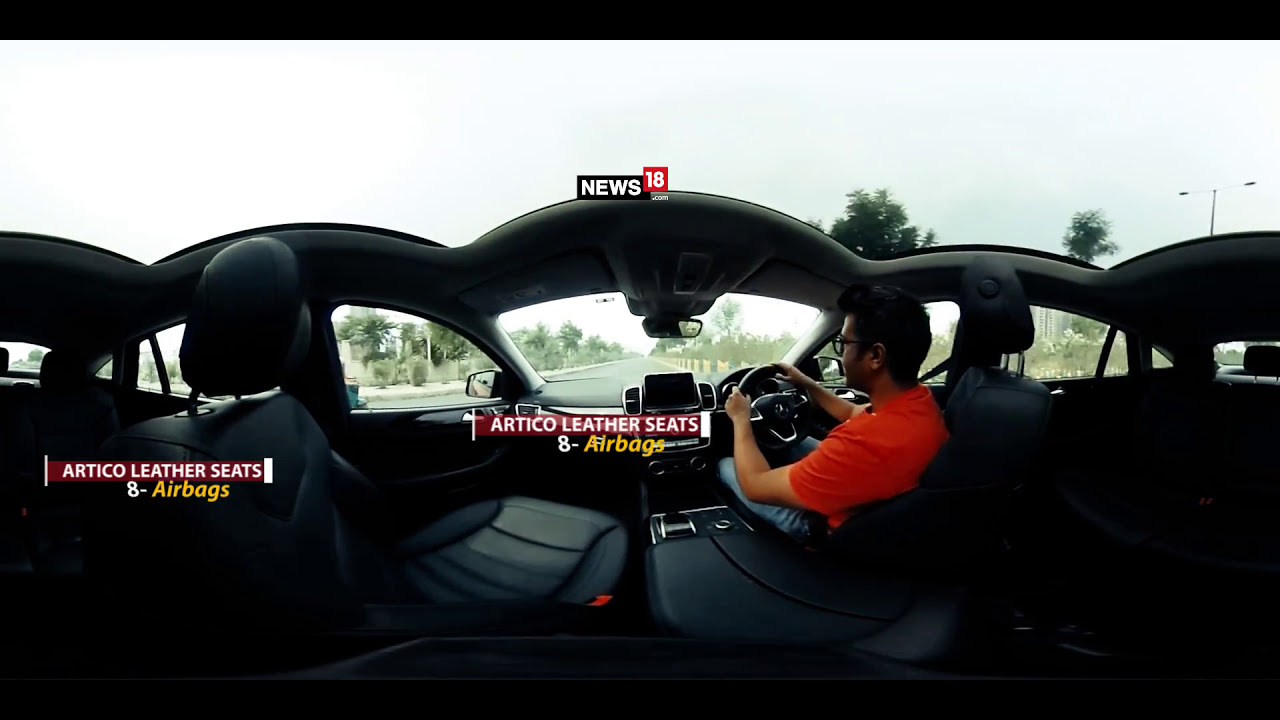This is a panoramic image of the interior of a car, capturing a unique, almost distorted perspective as if seen from multiple viewpoints inside the vehicle. A man with very dark hair, wearing dark-framed glasses and an orange short-sleeve shirt, is seated at the steering wheel on the right side. The car's interior is black, and the rear seats appear to be facing the passenger seats, adding to the unusual view. The scene outside the car includes visible palm trees, bushes, a road, and a sidewalk, along with a streetlight on the right side.

Prominently displayed above the image is the "News 18" logo, with "News" in white font inside a black rectangle and "18" in white within a red square. This branding suggests the image might be a still shot from a news video, possibly covering automotive topics like racing. Inside the car, repeated text in white, red, and yellow fonts highlights features such as "Artico Leather Seats" and "8 Airbags." These phrases are visible near the steering wheel and again on what seem to be the swiveled seats, reinforcing the emphasis on the car's interior features.